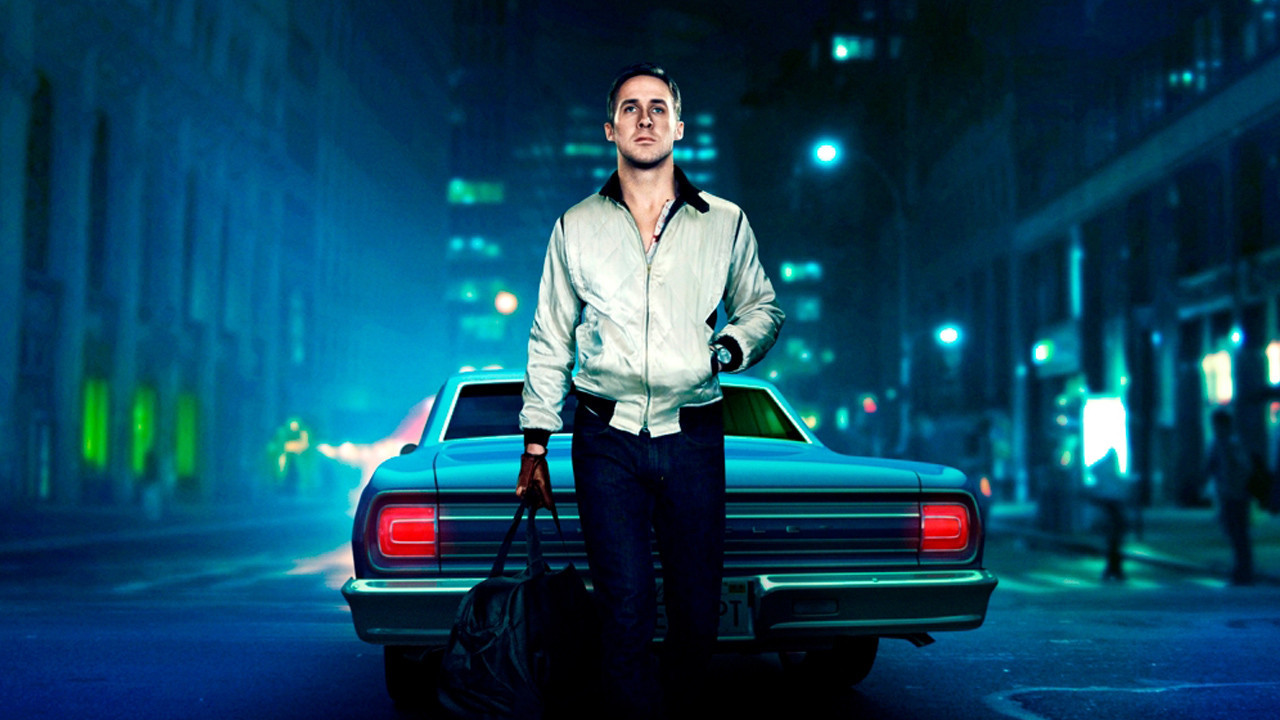In this nighttime image, a man resembling actor Ryan Gosling stands in the center of a dimly lit city street, surrounded by high-rise buildings illuminated with a blue tint. He sports a white bomber jacket with a black collar, dark blue jeans, and brown gloves. His left hand is tucked into his jacket pocket while his right hand holds a black leather duffel bag. Behind him is a vintage blue car, possibly a Chevrolet or Chevelle, oriented in the opposite direction. The street is lined with buildings on both sides, some with lit windows, especially on the lower floors where green lights are visible. The scene, reminiscent of a cinematic or video game setting, has a gritty, digital quality, enhanced by sparse street lighting and the ambient glow from the surrounding architecture. Another person is faintly visible in the background to the right, contributing to the urban atmosphere.